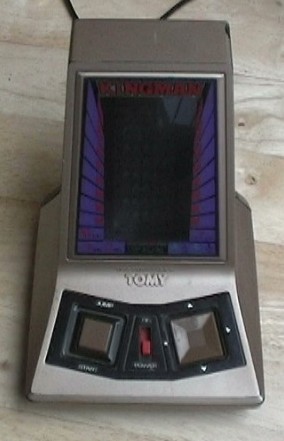This photograph is an overhead close-up view of a device placed on a light gray wooden surface. The device features a silvery gray base, likely plastic or metal, with a prominent square button, a non-functional switch, and a silver indentation bordered by black. Centered on the base are raised gray letters spelling "T.O.M.Y." Atop the base, a brown box extends upwards, housing two dark brown antennas. Above this box, there is a blue rectangular area with horizontal dark blue stripes and a central gray and black section. The red letters "KINGMAN" are inscribed at the top of this blue area. The device includes several switches: a red on-off lever, currently in the down position, and a brown button surrounded by white writing. Another square, lighter brown box on the device features white arrows at its corners.